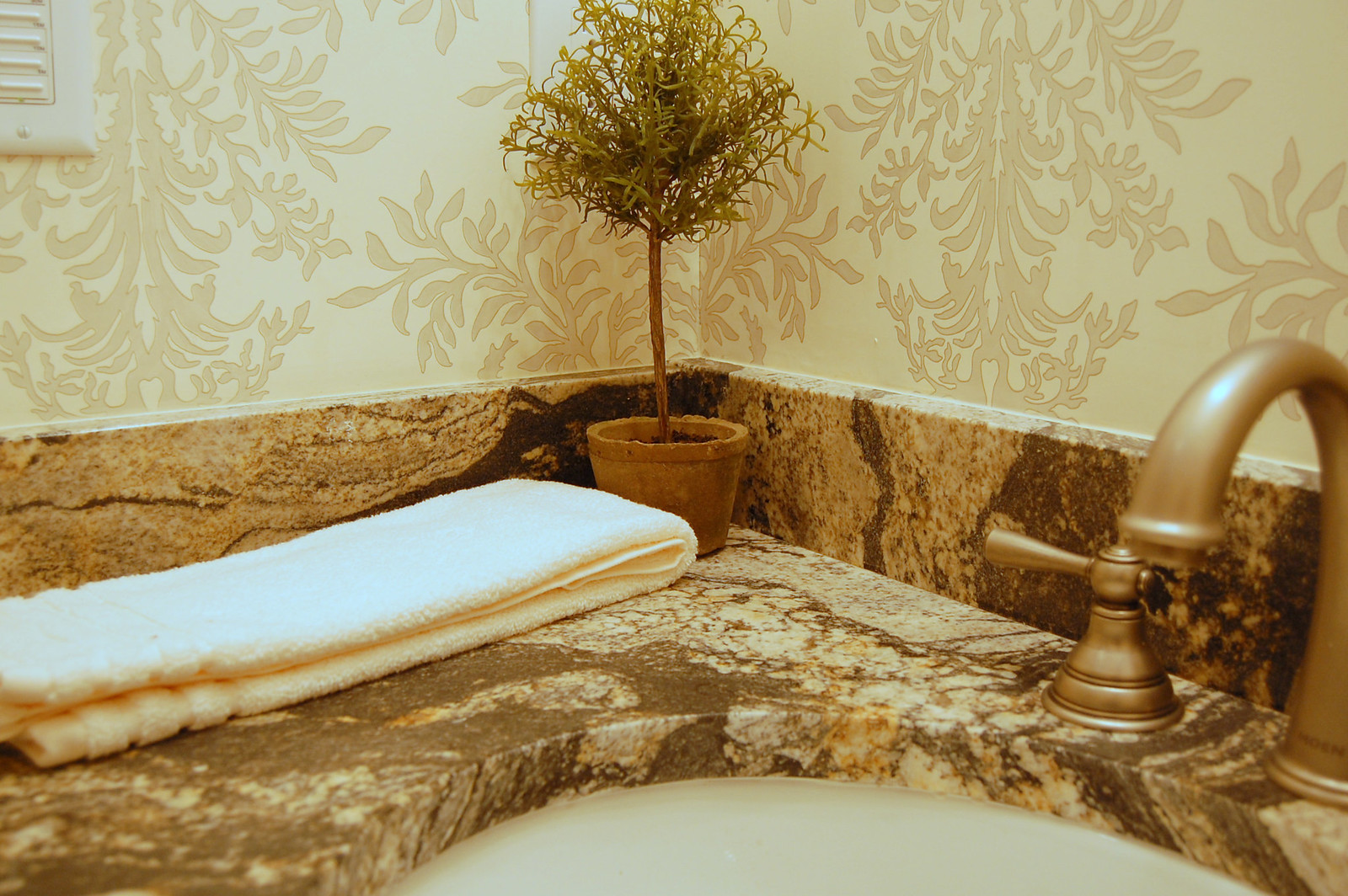The image presents a meticulously arranged bathroom corner with an artistic flair, possibly enhanced by a sepia tone filter. Dominating the frame is a close-up of a sink with a pale bronze hue, though this coloration might be the result of the filter. The viewpoint captures only the spigot and the left handle of the sink, omitting the right handle from the composition.

Adorning the countertop, which extends partially up the wall and is crafted from brown and white marble, a neatly folded white hand towel adds a touch of elegance. Adjacent to the towel, a plant rests in a terracotta pot, though its health appears questionable as its pale green, spiky leaves suggest distress. The plant could be perceived as a miniature tree.

The background features an art deco-inspired wallpaper, characterized by a repeating leaf-like pattern in shades of cream and darker cream, mirroring the natural element depicted by the potted plant. A white vent with a closed screw is partially visible in the top left corner of the image, hinting at a meticulous and orderly setting.

The sink basin, from what little is visible, appears to be a creamy white, contributing to the overall pristine and sophisticated atmosphere. The scene likely depicts a high-end bathroom, either in an upscale hotel or a meticulously maintained home, reflecting an appreciation for cleanliness and style.